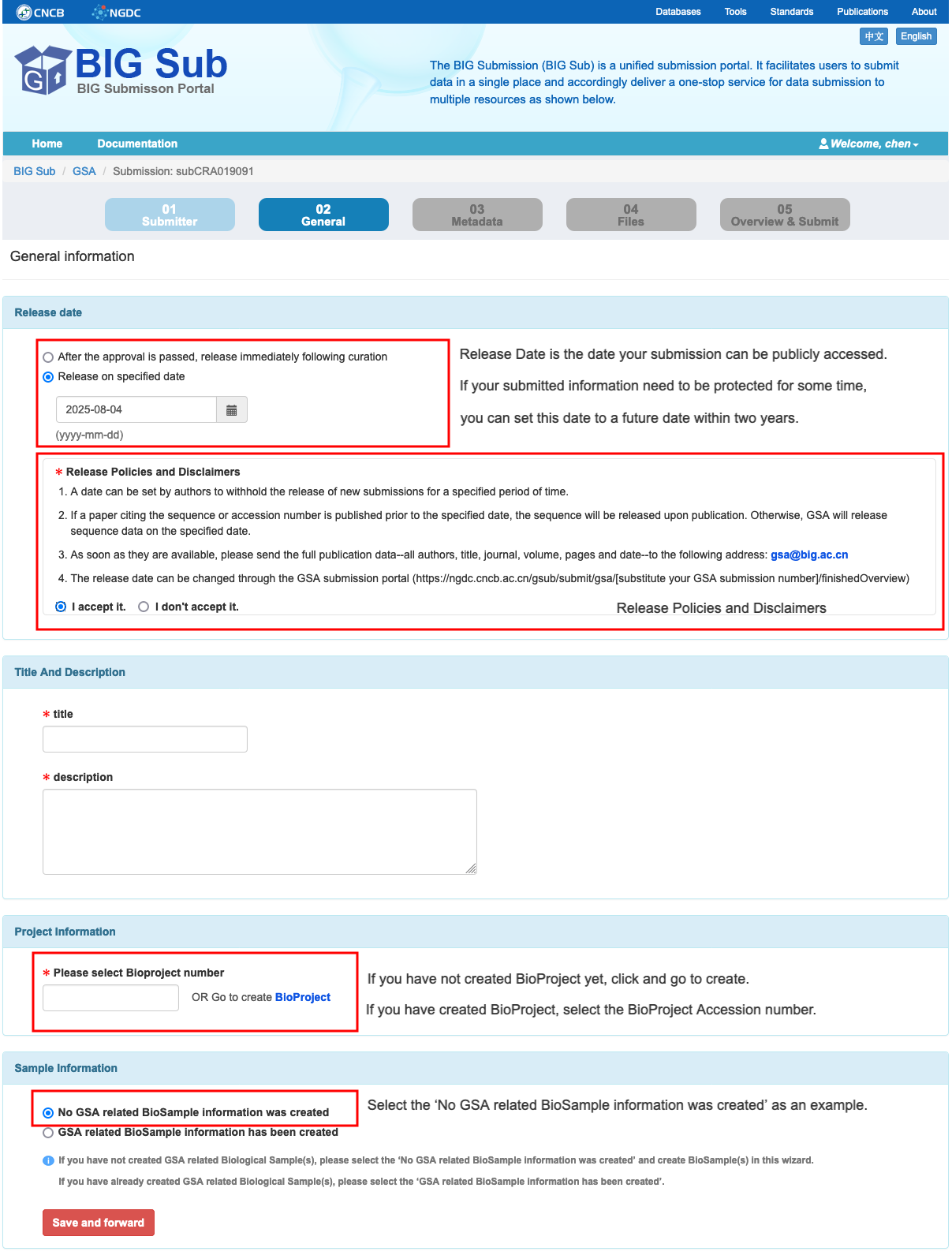**Detailed Caption:**

The image showcases a lengthy webpage of an application or a website, specifically a form interface titled "Big Sub, Big Submission Portal." The header indicates that "Big Sub" is a unified submission portal designed to facilitate users in submitting data efficiently in one place. It provides a comprehensive one-stop service for data submission across multiple resources.

Below the header, a five-step process illustrates the submission workflow:
1. **Submitter 01 (Current Step)**: This is the step currently active, indicated by its title "General."
2. **Metadata**: This step is yet to be completed.
3. **Files**: Another forthcoming step.
4. **Overview and Submit**: The final step before submission.

The central section of the form contains detailed fields under the heading "General Information." Users are required to input the "Release Date," with options to select a specific date, release immediately following the approval and curation process, or release on the approval date. An explanation clarifies that the "Release Date" is when the submission will be publicly available.

Users must accept or reject the release policies and disclaimers to proceed. The form includes empty fields for "Title" and "Description." There is a section for "Project Information" where users can either select from provided options or enter a "Bio Project Number."

However, a red box highlights a warning stating, "No GSA-related bio sample was created," under the "Sample Information" section.

At the very bottom of the form, a red button labeled "Save and Forward" is available for users to save their progress and move to the next step.